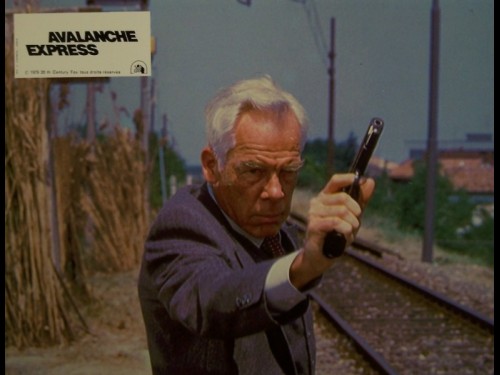This image appears to be a still from a very old movie, likely from the 1960s or 70s, with potential ties to a western or action genre. At the top left-hand corner, there's a card that says "Avalanche Express" accompanied by a small logo. The main focus of the image is an older man with gray hair, wearing a dark blue or medium gray suit with a white undershirt and cuff, holding a handgun pointed skyward with a determined expression on his face. He is standing on a stone or rocky ground surface, in front of train tracks that cut through the center of the image. Behind him, we see a mixture of industrial and natural elements—there's a factory-like building on the right, several telephone poles, sparse vegetation, and what appears to be stacks of wood or hay to the left. The sky is faded, appearing either dark blue or light gray, suggesting an outdoor scene possibly set in the fall. The man is positioned centrally, enhancing his prominence as the focal point of this intriguing and nostalgic composition.